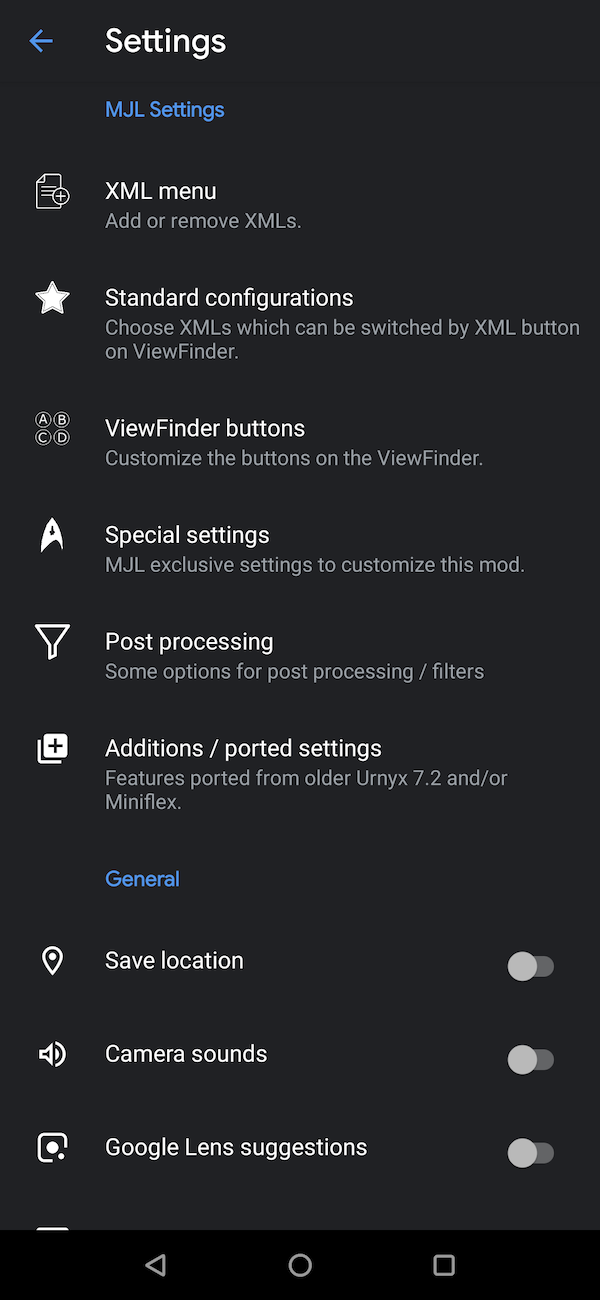The image depicts an iPhone with a black background, specifically displaying a settings menu. The top of the screen features the title "Settings," centered, with a back arrow to its left. Directly below this title is the section labeled "MJL Settings," indicating perhaps the owner's initials, with these letters in blue.

Following that is the "XML Menu" option, tagged with "Add or remove XMLs." Beneath this is "Standard Configurations," providing the ability to choose XMLs that can be switched via the XML button on the viewfinder. Accompanying this text is a filled-in white star icon to the left. Under "Standard Configurations," there is a section titled "Viewfinder Buttons," instructing users to customize the buttons on the viewfinder, marked by four dots labeled ABCD to the left.

Next, the menu lists "Special Settings," identified by an arrow icon to the left. Under this heading, it specifies "MJL exclusive settings to customize this mod." Below this, another heading "Post Processing" appears, with options for post-processing/filters, accompanied by a funnel icon to the left.

Finally, the "Additions" section notes "Ported settings" featuring elements from older UMYX 7.2 and/or Miniflex versions. The word "General" is highlighted in blue, and under this category, the options listed are "Save Location," "Camera Sounds," and "Google Lens Suggestions." Each of these options has a corresponding switch to toggle the feature on or off, with an icon to the left representing each option.